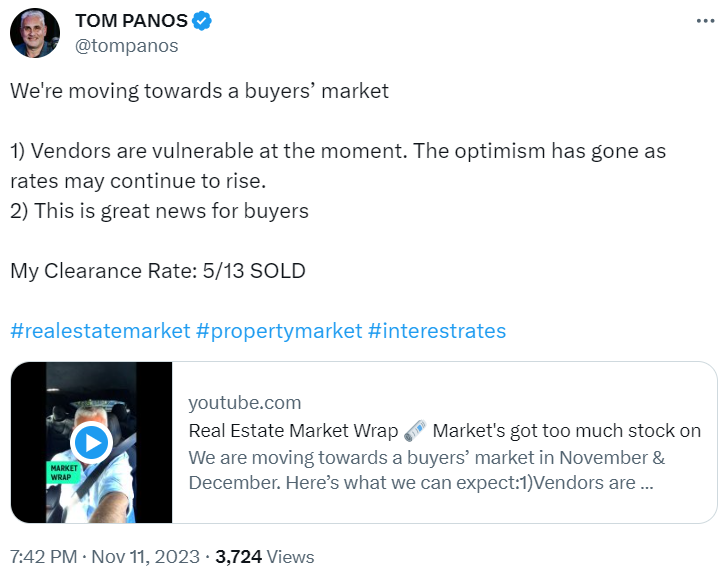Screenshot of a tweet by Tom Panos, displaying his verified account (blue checkmark) with the handle @TomPanos. His profile picture, situated to the left, features a circular image of a man with short, white hair. 

The tweet reads: "We're moving towards a buyer's market," followed by a numbered list:

1. Vendors are vulnerable at the moment; the optimism has gone as rates may continue to rise.
2. This is great news for buyers.

The tweet also mentions, "My clearance rate: 5 out of 13 sold," and includes three hashtags in blue text: #realestatemarket, #propertymarket, and #interestrates.

Embedded below the tweet is a snippet linking to a YouTube video. The thumbnail is on the left and the accompanying text on the right reads: "youtube.com, Real Estate Market Rap: Market's Got Too Much Stock On."